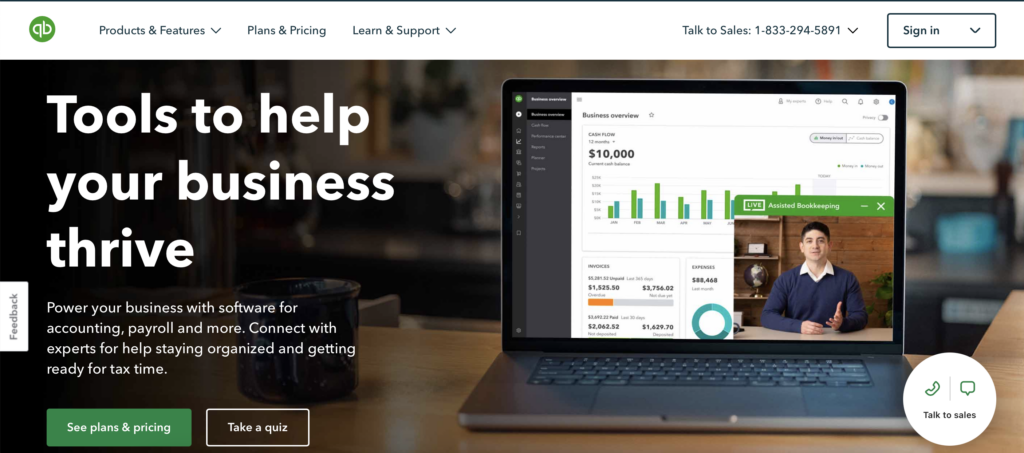The website features a clean white header bar with navigation links starting from the left: "Product and Features" with a drop-down menu, "Plans and Pricing," and "Learning and Support" with another drop-down menu. On the right side of the header bar, there are options to "Talk to Sales" with the number 1-833-294-5891 and a drop-down menu, and "Sign In" accompanied by a drop-down as well.

Just below the header is a central image of a laptop resting on a desk. The laptop screen displays various sales information, including a prominent figure of $10,000 and several bar graphs, with a person featured in the interface. 

Dominating the left side of the image in bold white text, the headline reads, "Tools to help your business thrive." Beneath this, in smaller white text, it states, "Power your business with software for accounting, payroll, and more. Connect with experts for help staying organized and getting ready for tax time."

Further down, there are two prominent buttons: a green button with white text that says "See Plans and Pricing," and next to it, a white-outlined button with white text that reads "Take a Quiz."

Lastly, on the lower left side of the page, a tab extends outward labeled "Feedback."